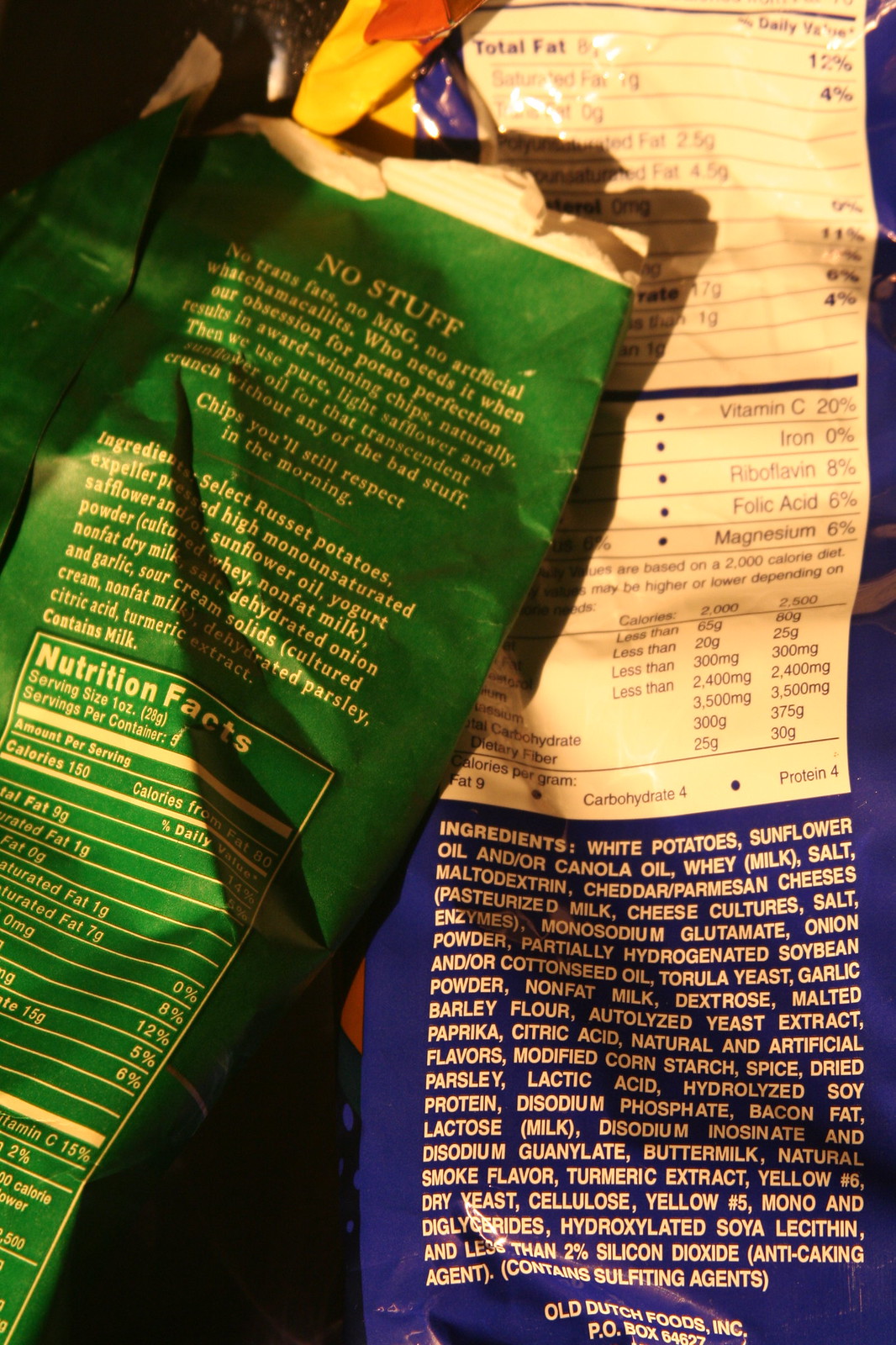The image features the back of two bags of potato chips, positioned side by side against a dark black background that provides minimal detail. The bag on the left is green and partially crumpled, displaying a notable white nutrition label. Key readable text includes "No Stuff," "No trans fats, no MSG, no artificial whatchamacallits," emphasizing a commitment to natural ingredients and quality. The green bag further details the use of pure light safflower and sunflower oil for a crunch without undesirable additives, promising "Chips you'll still respect in the morning." The product description is complemented by an ingredients list with "select russet potatoes" as the first item, though some words are somewhat obscured.

The bag on the right is dark blue and appears flat or empty, with a nutritional panel in pale yellow and orange towards the top that resembles a bag clip. The ingredient list is printed in white text on the blue background, with "white potatoes" as the primary ingredient. The visible part of the label mentions Old Dutch Foods Incorporated and a P.O. Box number 64627, indicating the manufacturer. The nutrition facts on both bags are standard, though they are partially cut off, making it difficult to see the complete information.